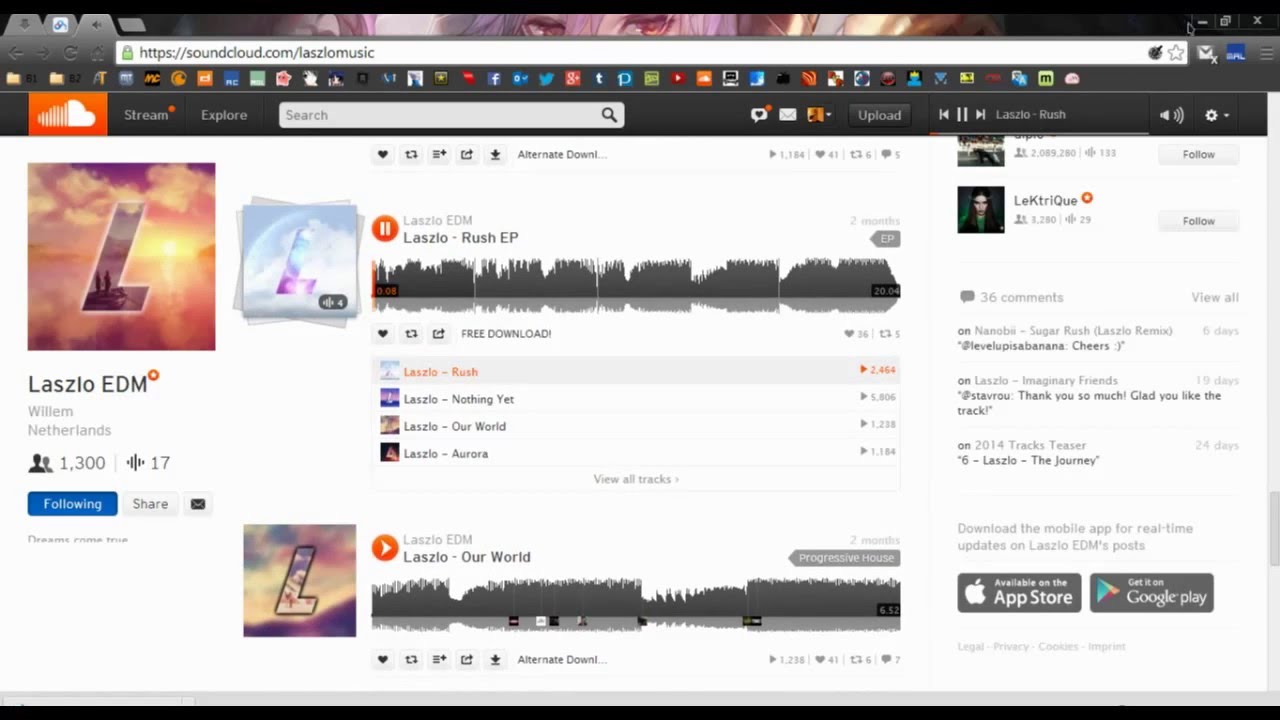This detailed screenshot captures a SoundCloud webpage viewed in a browser window with a visually striking animation-themed background featuring a character’s eyes amid various shades of purple. The URL displayed in the address bar reads "SoundCloud.com/LazloMusic."

At the top-left corner of the page, the distinctive SoundCloud logo is showcased as an orange rectangle containing a cloud, where one half is entirely white and the other half is white adorned with horizontal, vertical orange lines. Below the logo, the website title reads "Lazio EDM," accompanied by cover art that is a square photograph depicting either a sunrise or sunset with a blend of beautiful yellow, pink, and purple hues. The letter "L" is prominently displayed in the center of the image, created from slightly different shades of purple that blend seamlessly with the background colors, indicating it's part of the photo.

The central part of the page features the primary SoundCloud player, set against a white background. The player displays the "Lazio Rush EP" title above the sound wave visualization. On the right side of the player, under a small photo of a woman with long brown hair, the name "LEKTRIQUE" (spelled "L-E-K-T-R-I-Q-U-E") is shown, accompanied by a gray "Follow" button.

In the lower-right corner, there are icons for downloading the SoundCloud mobile app, including a gray rectangle with the Apple logo for the App Store and another with the colorful Prism logo for Google Play.